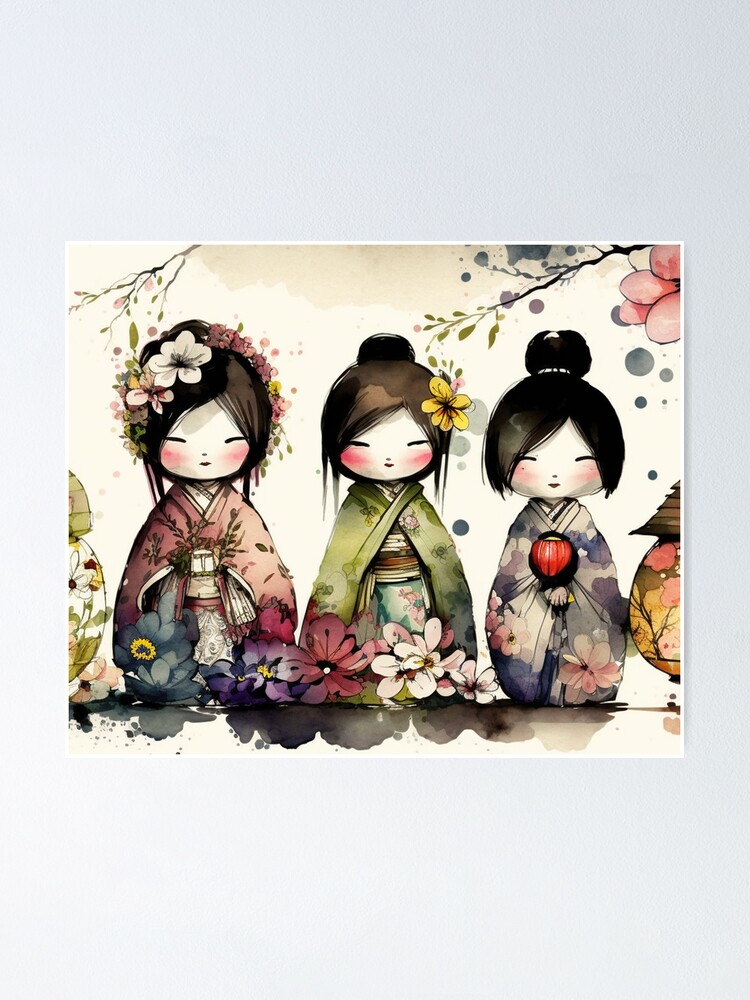This vibrant, rectangular artistic print, set against a subtly gradated blue-to-gray background, captures a whimsical and colorful interpretation of three Asian-inspired dolls, possibly Japanese or Chinese, resembling traditional figures. Each doll has strikingly similar, dark brown-black hair, parted at the middle with a slight fringe, styled into buns at the back. The doll on the left, dressed in a pink robe adorned with a floral pattern and white undergarments, holds a plant and has an elaborate hair adornment featuring a large white flower and a smaller pink one. The central doll, distinguishable by a single yellow flower in her hair, wears a green robe with a decorative undergarment in shades of turquoise and reddish hues. The rightmost doll dons a dark violet robe with pink floral details, hinting at traditional kimono influences, and has a more abstract, colorful floral pattern beneath. These dolls, each with tiny slit eyes, small mouths, and dot-like noses, are set amidst a foreground blooming with pink and turquoise flowers, mirroring the intricate floral arrangements in their hair and robes. Above them, branches with green leaves add a touch of nature. To the lower right, a traditional paper lamp with floral motifs, partially visible, complements the serene and picturesque composition, capturing the delicate and detailed beauty of this unique piece.